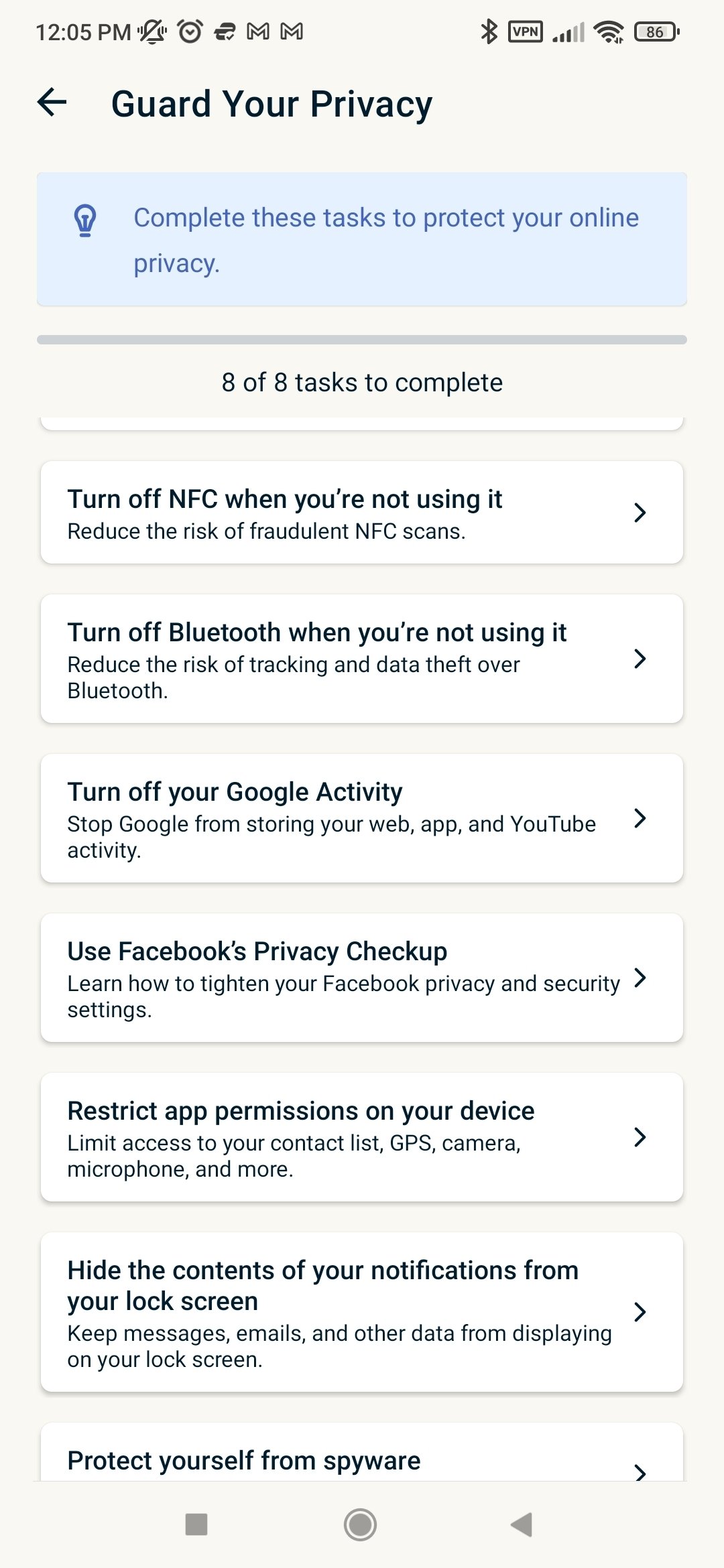Screenshot of Privacy Settings Page: A Detailed Description

The screenshot displays a beige-colored settings page titled "Guard Your Privacy" in bold black text at the top. On the left of the title, a back arrow button is visible, allowing users to return to the previous menu. Directly below this title, a prominent blue box with a lightbulb icon to the left contains the text "Complete These Tasks to Protect Your Online Privacy."

Underneath the blue box, a gray line divider separates it from the subsequent content. Following this divider, there is a heading stating "8 of 8 tasks to complete," indicating the user's progress in completing privacy-related tasks. The listed tasks include both a title and an explanation beneath each, with a forward arrow to the right of each task, potentially for navigating to further details.

The listed privacy tasks are:
1. **Turn off NFC when you're not using it** – Disable Near Field Communication to enhance privacy.
2. **Turn off Bluetooth when you're not using it** – Switch off Bluetooth to prevent unauthorized access.
3. **Turn off your Google activity** – Stop Google from tracking your online actions.
4. **Use Facebook's Privacy Checkup** – Review and manage your Facebook privacy settings.
5. **Restrict app permissions on your phone** – Limit what apps can access on your device.
6. **Hide the contents of your notifications from your lock screen** – Prevent sensitive information from appearing on your lock screen notifications.

This detailed descriptive caption encompasses all elements seen in the screenshot, providing a comprehensive understanding of the image's content.